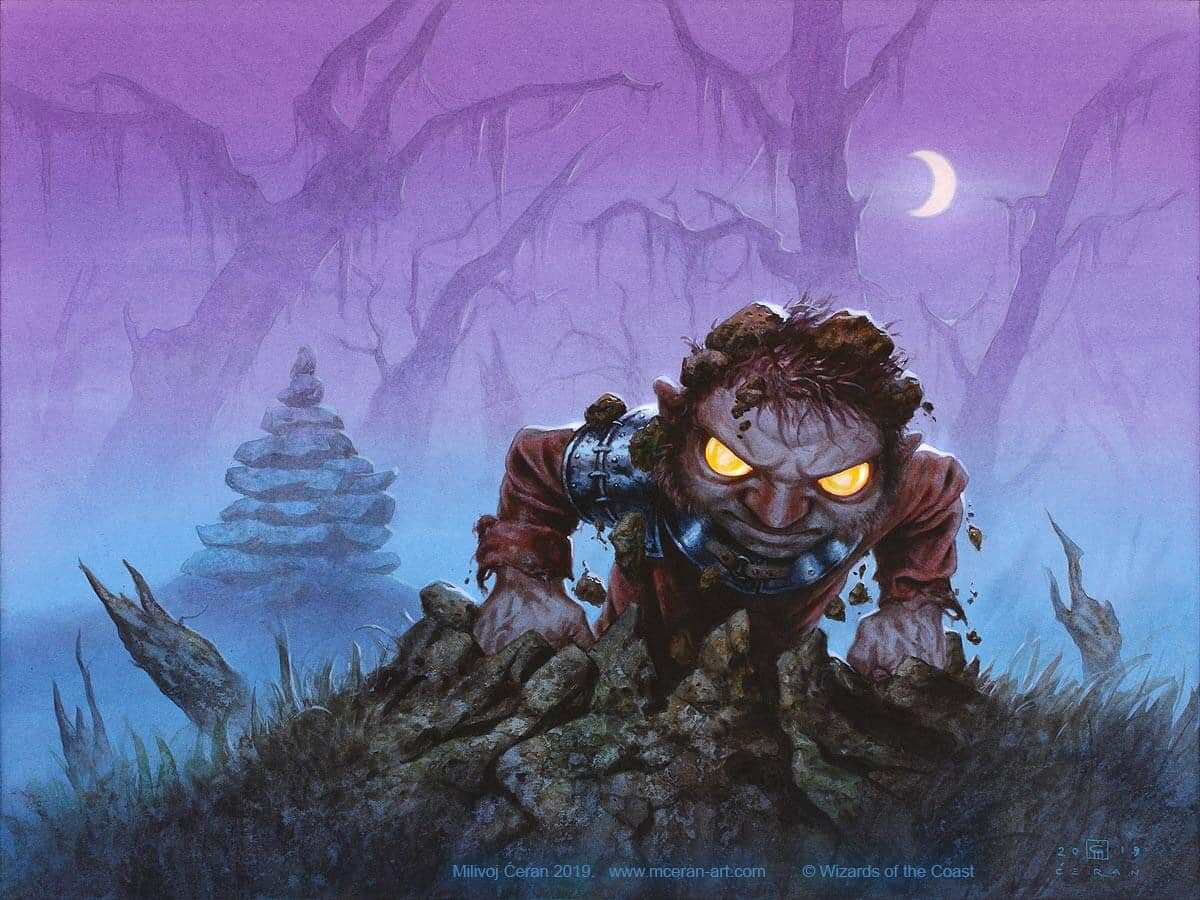The digital illustration depicts a small grassy hill crowned by crumbling rocks from which a creature is emerging. The creature resembles a hobbit-like troll or a Smeagol with hair, and it is clothed. Its large, angry yellow eyes, half-circles in shape, convey a menacing expression. The creature's skin is a peachy white color, and it has reddish-brown hair. It wears a long-sleeved reddish shirt and a metal plate around its neck that extends to its chest. Only the upper half of its body is visible as it pushes itself out from the rocks with clenched fists pressing against the ground.

Behind the creature lies a dead forest, with spooky tree silhouettes fading into the night sky. A crescent moon hangs in the top right corner, while a pile of rocks sits to the creature's left. The sky features a gradient blend of purple and blue hues, with a misty effect surrounding the creature, and the entire image is overlayed with a grainy texture.

At the bottom center of the image, text reads "Milevaj Saran 2019 www.mceran-art.com © Wizards of the Coast." In the bottom right corner, small, indistinct symbols line up, with a discernible "2," "9," and several other arcane symbols.